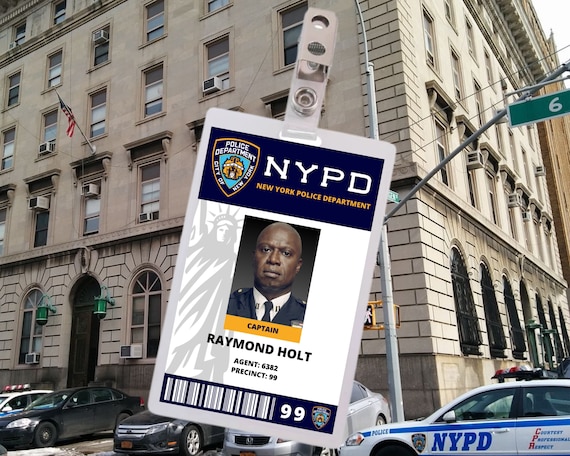The image appears to be a promotional screenshot from the television show "Brooklyn 99." The background features a multi-story, concrete-beige building that resembles a police headquarters, with distinctive arch doorways and windows on the first floor, likely suggesting a New York setting. Several NYPD police cars and some pedestrian vehicles are parked beside the building, with an American flag visible atop the structure, indicating it might be during the day.

Prominently overlaid in the foreground is a large NYPD police badge. This badge includes the NYPD shield emblem, and a detailed ID section featuring a formal photograph of Captain Raymond Holt, a bald man in uniform. Below his picture, within an orange rectangle, the title "Captain" is displayed, followed by his name "Raymond Holt" in black font, agent number "6382," and "Precinct 99." The ID also bears a blue rectangular border with white line designs reminiscent of a barcode, again showcasing the number 99 alongside another police shield emblem. Additionally, a nearly translucent image of the Statue of Liberty is subtly embedded within the badge’s background, adding depth and a New York vibe to the graphics.